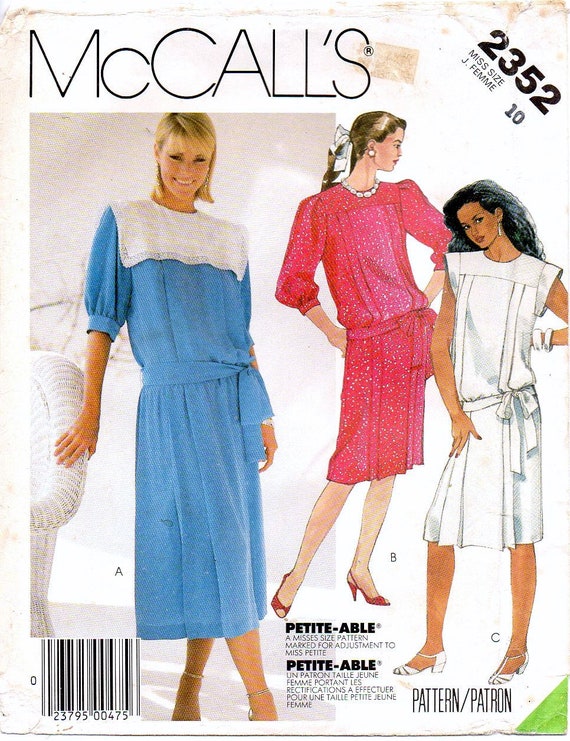This image is an old, slightly tattered McCall's sewing pattern advertisement, numbered 2352, meant for "Miss Size J, Female 10." The pattern is laid on a white background and shows some signs of wear, including edge staining and remnants of a price sticker. 

In the upper right corner, "2352 Miss Size J Female 10" is printed prominently. The bottom left corner features a barcode labeled 2379500475. The bottom middle displays the text "Petite Pattern/Patron."

The image features three women. On the left is an actual photograph of a blonde woman with shoulder-length hair and bangs, dressed in a blue knee-length dress. The dress has a white, lace-edged square collar overlay and sleeves that reach the elbow, ending in cuffs. She wears strappy sandals, a sash at the waist, and stands slightly looking down, with her right hand resting on a piece of white wicker furniture.

Next to her are two illustrations. One is a red dress with three-quarter-length sleeves. The other shows a black woman in a sleeveless white dress with small cap sleeves and no collar overlay. This comprehensive visual representation depicts the styles conveyed by this vintage sewing pattern.